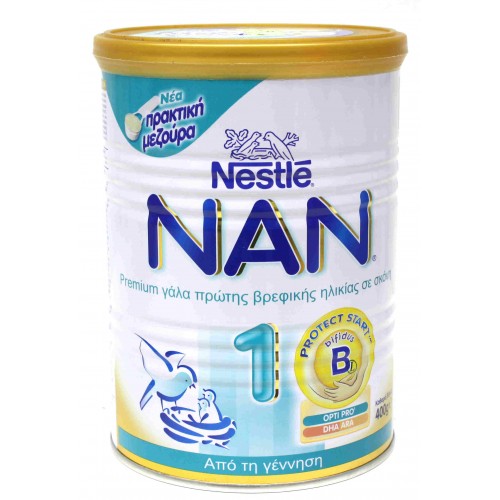The image depicts a can of baby formula from the brand Nestlé. The front of the can is predominantly white, with additional coloring details including blue in the middle and yellow accents on the top and bottom. The Nestlé logo, situated at the top, features two blue baby birds in a nest being looked after by a parent bird, all surrounded by leaves and branches. Under the Nestlé logo, the product name "NAN" is displayed prominently, accompanied by the word "Premium" and some foreign text, which appears to be in Russian and consists of six words. A notable detail is the number "1" displayed in an aquamarine hue, indicating it's the first stage of the formula. Additionally, on the right side of the can, there's a yellow circle containing the blue text "Protect Start" and the word "Bifidus," alongside "DHA" and other Russian words. Lastly, in the upper left corner, there's an illustration of a scooper with a white powdery substance, further suggesting that this is indeed baby formula.